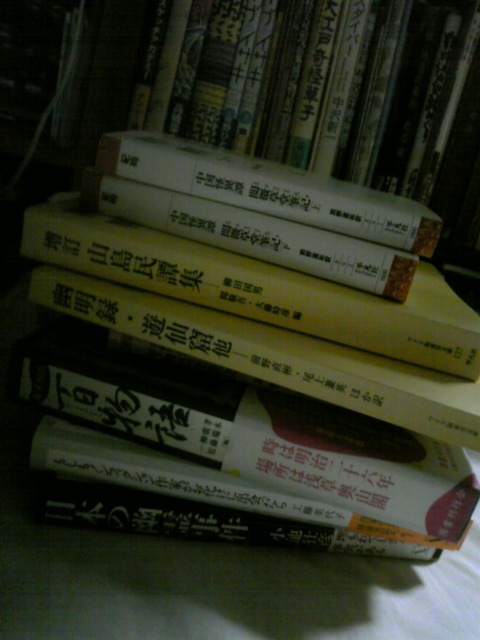The image depicts a portrait-oriented, dark photograph of a stack of seven books, organized from largest at the bottom to smallest at the top, all resting horizontally on what appears to be a white cloth or table. The spines of the books, each featuring Japanese or Chinese characters, are prominently facing the camera, with the top edge of each book to the left side and the bottom edge to the right.

The top two books in the stack are white with black lettering. Below them are two yellow-bound books, also with black lettering. Following the yellow books is a dark one, and beneath it, another white book bearing black and red lettering on its spine. Finally, the book at the base of the stack has a black spine with white text. 

In the background, an additional set of vertically stacked books is visible on a bookshelf, casting shadows and illuminated by backlighting, further enhancing the composition's depth and contrast.